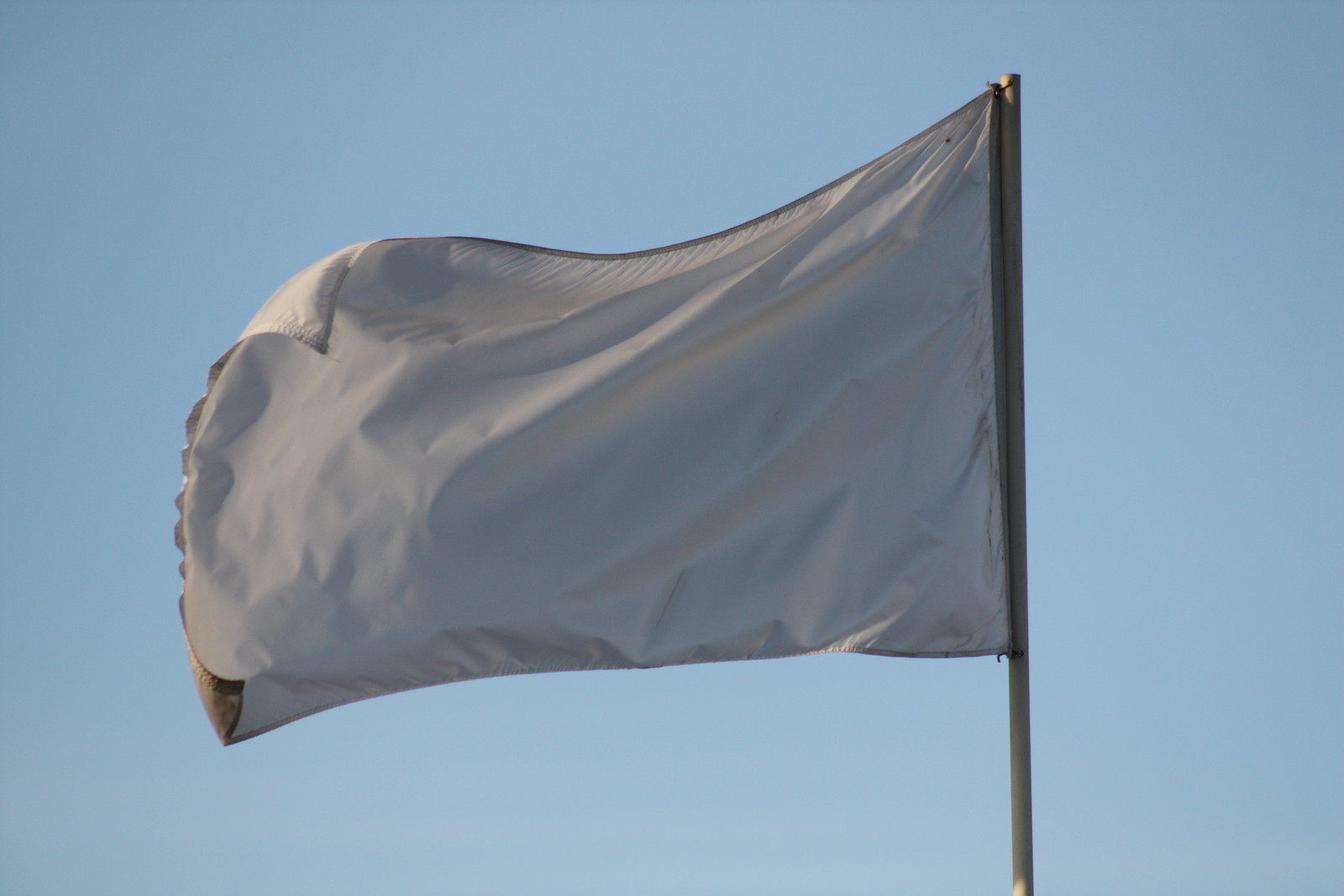A photograph taken outdoors during the daytime shows a white or extremely light gray flag waving in the breeze against a grayish blue sky. The flag is attached to a white flagpole, visible on the right side of the image, which is rectangular and wider than it is tall. The sky appears plain with no clouds, accentuating the movement of the flag.

The flag itself is simple, with no logos or images on its visible side. Its corners are curling and overlapping due to the wind, creating ripples and a dynamic flow in the fabric. The left edge of the flag, furthest from the pole, appears slightly serrated and ruffled. Near the bottom left corner, where the flag curls over, there is a hint of a brownish shadow, possibly indicating dirt or a darker edge on the opposite side. The motion of the flag and the breeze create light and shadow play, adding texture to the otherwise smooth fabric.